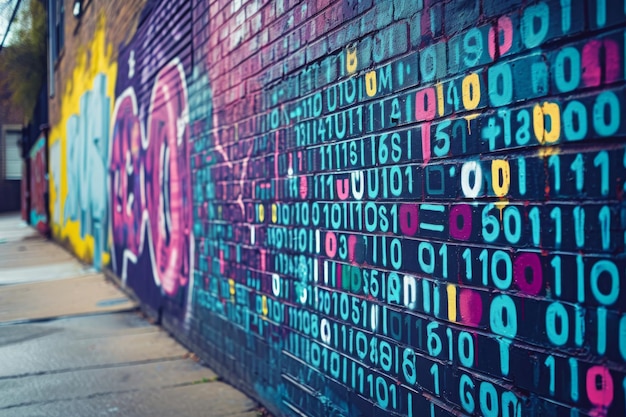This photo captures an external view from the street side, focusing on a brick wall drenched in colorful graffiti. The brick wall, likely part of an alleyway, is decorated with a myriad of vivid colors and distinct graffiti styles. The most prominent graffiti, closest to the camera, is an intricate matrix of numbers resembling binary code, featuring a mix of zeros, ones, sixes, and fives in various hues of blue, yellow, and purple. This section features a dark blue background with the numbers primarily in aqua, pink, and light blue. Further down the wall, the graffiti transitions into more abstract and colorful drawings, blending shades of purple, pink, yellow, and blue, though the details blur as the perspective recedes into the background. The sidewalk at the bottom left of the image adds a diagonal touch in beige, subtly contrasting with the vibrantly adorned brick surface. At the vanishing point of the alley, another building is faintly visible.